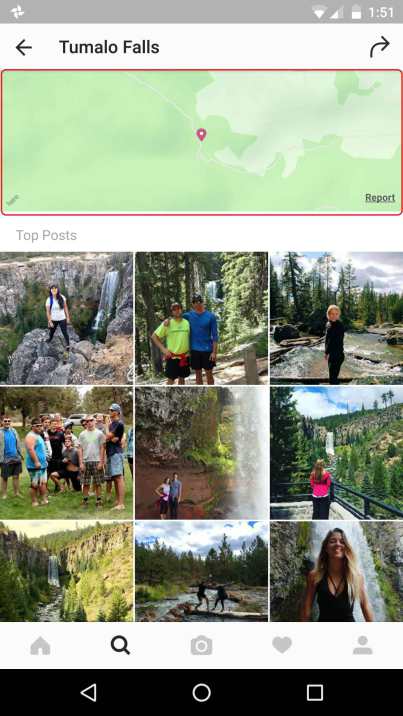Screenshot Description: Google Page for Tumalo Falls

This screenshot captures a Google search page dedicated to Tumalo Falls, presented on a white background. At the top, the page title "Tumalo Falls" is prominently displayed in bold black font. To the left and right of the title, there are navigation arrows: a left-pointing arrow and a right-curving arrow, respectively.

Below the title, the page features a sizable map with a red-outlined box highlighting the location of Tumalo Falls. A pin marks the exact spot of the falls on the map.

Further down the page, a section labeled "Top Posts" showcases images taken by visitors at Tumalo Falls. This section contains nine thumbnail photos arranged in a 3x3 grid, displaying three rows of three images each.

At the bottom of the screenshot, the navigation bar includes five icons: a home button, a search button, a camera icon, a heart icon, and a person icon. Finally, at the very bottom, part of the phone’s control panel is visible, featuring a triangle pointing left for back navigation, a circle for returning to the home screen, and a square icon.